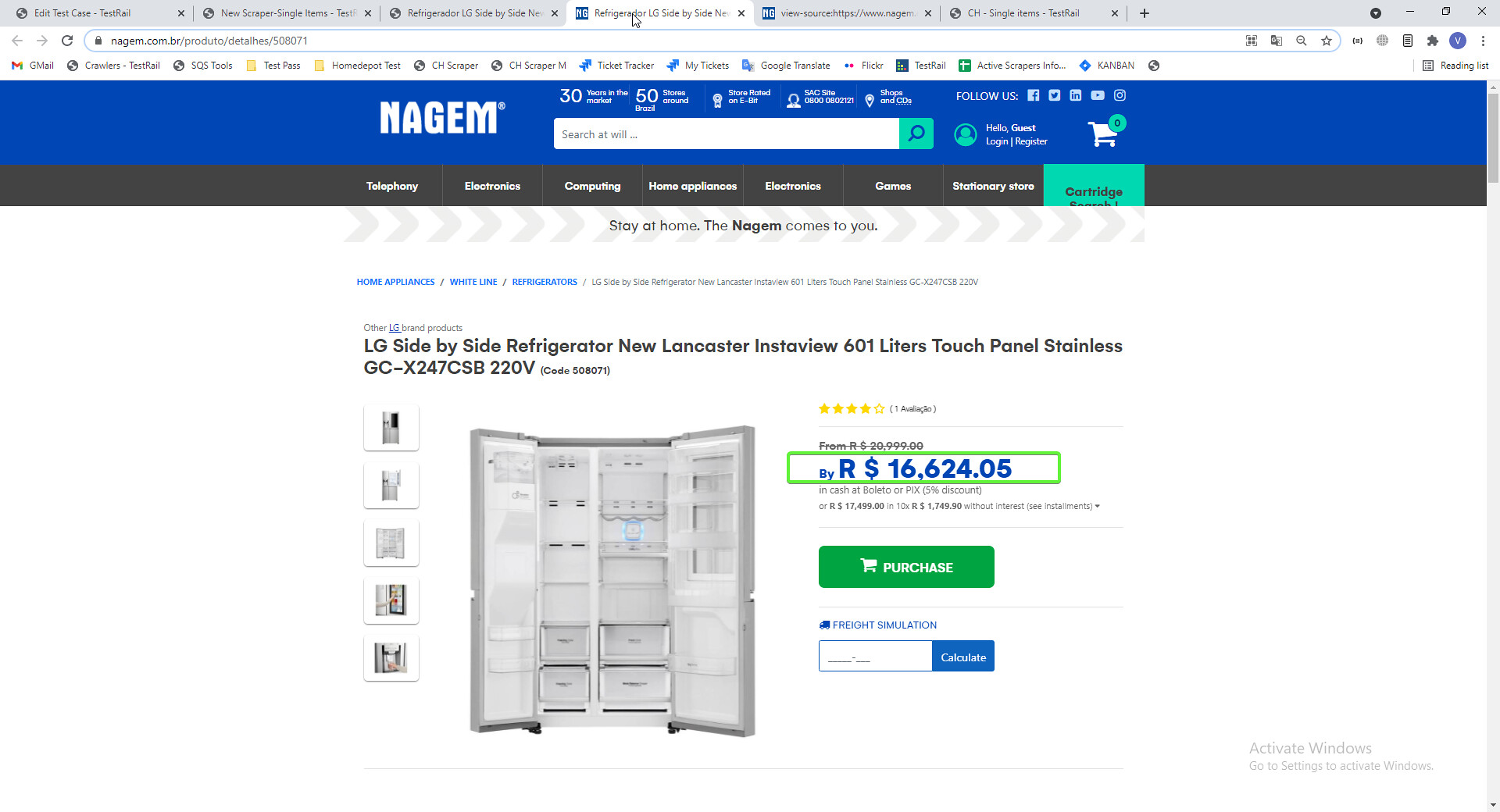This image is a color photograph of a computer screen displaying a webpage on an online shopping site named "N-A-G-L-E-M" (with a trademark symbol). The screenshot is from a Chrome or Firefox web browser with six tabs open at the top. The webpage features a detailed product listing for an LG Side-by-Side Refrigerator, specifically the New Lancaster InstaView model with a 601-liter capacity, a touch panel, and a stainless steel finish (model number GC-X247CS-B220V). The price is listed as 16,624.05 Brazilian Reais.

At the top of the webpage, there is a dark blue banner with a search bar and the N-A-G-L-E-M trademark logo. Above this banner, it reads "30 years of the market, 50 stores around Brazil, store rated on e-list, SAC site with some illegible numbers, shoes and CDs" followed by social media icons linking to Facebook, Twitter, Instagram, YouTube, and LinkedIn. The site features a white shopping cart icon displaying '0' items next to a "Hello Guest, Log in, Register" prompt with a generic user icon.

The navigation bar includes categories like Telephony, Electronics, Computing, Home Appliances, Electronics, Games, Stationary Store, and Cartridge, with a subtitle below stating "Stay at home. The login comes to you." The product section prominently shows the white refrigerator with its doors open, revealing several drawers. To the left of the main image, there are additional click-through views. To the right, it shows a four-star rating, the price, a green purchase button, and a freight simulation calculator.